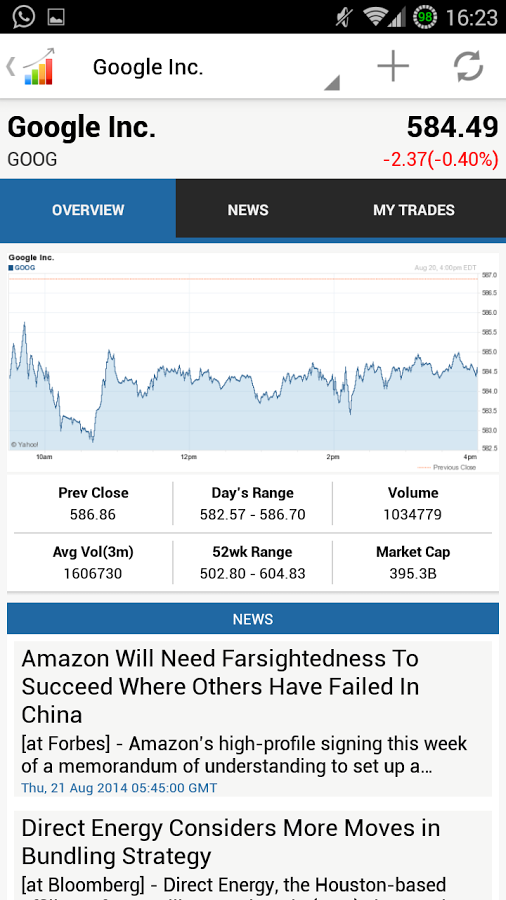A detailed caption for this image could be:

"The image depicts a black speaker with no visible markings or signals, except for a full Wi-Fi indicator and a 90% battery level displayed at 16:23. In the foreground, there is a colorful graph featuring blue, green, yellow, and red rectangles. On the graph, several labels are visible: a blue rectangle marked "Overview," a black rectangle labeled "News," and another black rectangle titled "My Trades." The graph also shows a timeline with indicators at 12 PM, 2 PM, and 4 PM. Additionally, it includes financial metrics: the previous closing price of 586.86, and current data with a figure of 584.49, down by 2.37 or 0.40%. Above the graph, there is a button labeled "Refresh" and a search bar indicating a query for "googling." The repetitive mention of the previous close emphasizes its significance in the presented financial data."